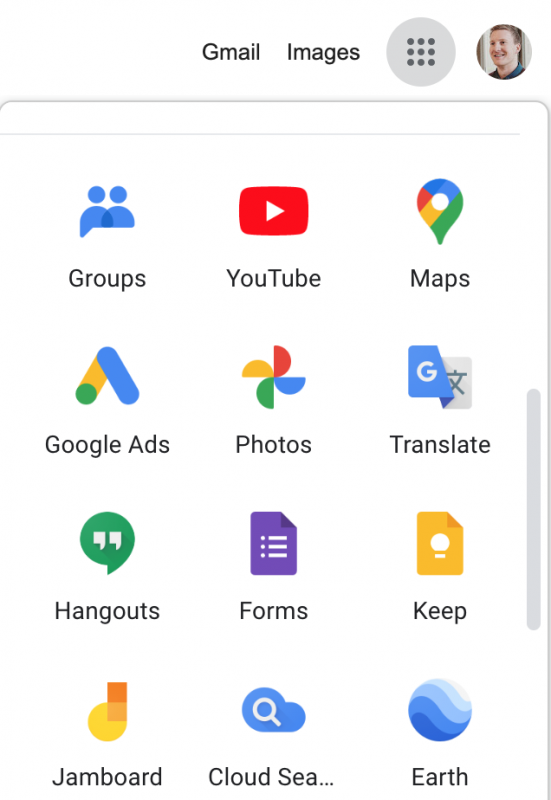This is a screenshot of a smartphone displaying a collection of Google apps. In the upper right-hand corner, there is a small profile picture featuring a young man with short blonde hair, wearing a collared shirt, and smiling. Next to his profile picture is a light gray circle containing nine dark dots arranged in a square, representing the app grid. Adjacent to these are the words "Gmail" and "Images."

Below this top row, the background is white and features four rows of three app icons each, with labels indicating the corresponding Google apps. Listed from left to right and top to bottom, the apps are:

1. Google Groups, represented by an icon showing two blue silhouettes of people.
2. YouTube, represented by a red square with a white play button (triangle) in the center.
3. Google Maps, represented by an icon with a colorful map pin.
4. Google Ads, represented by an icon with a blue, green, and yellow "A" symbol.
5. Google Photos, represented by a multicolored pinwheel icon.
6. Google Translate, represented by an icon combining a "G" and another language character.
7. Google Hangouts, represented by a green speech bubble with white quotation marks.
8. Google Forms, represented by a purple sheet of paper with lines.
9. Google Keep, represented by a yellow lightbulb icon.
10. Google Jamboard, represented by an orange "J" on a red and yellow background.
11. Google Cloud Search, represented by a blue magnifying glass encircling a cloud.
12. Google Earth, represented by an icon showing a stylized globe.